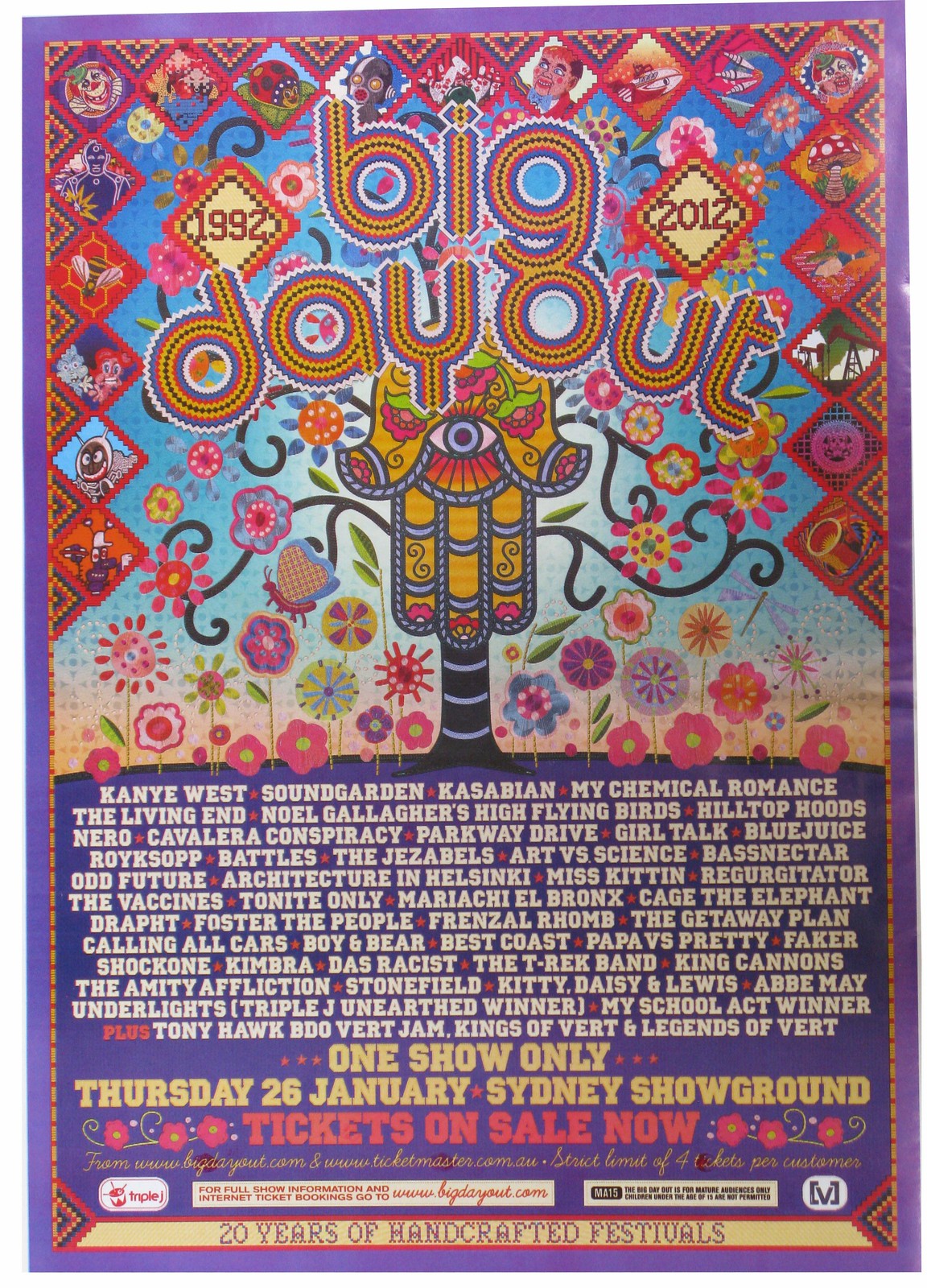This image is a rectangular concert advertisement, approximately six inches tall and four inches wide. It features a vibrant purple border enclosing the design. The background gradient transitions from light brown at the bottom to blue at the top. Around the edges, there are red, crimped-edge diamonds containing various cartoonish images.

At the center top of the advertisement, the title "Big Day Out" is prominently displayed, flanked by the years "1992" and "2012," indicating a 20-year celebration of the festival. Below the title, there's an intriguing illustration: a hand facing downward with an eye in its palm and a tree trunk extending from the bottom of the hand.

The lower section of the poster lists an array of musical acts against a purple background, with artist names in white text. Noteworthy performers include Kanye West, Soundgarden, Kasabian, My Chemical Romance, The Living End, Hilltop Hoods, Nero, and many others.

Additional details highlight the event specifics. In yellow text, it announces "One Show Only, Thursday, 26 January, Sydney Showground" and, in red, "Tickets on Sale Now." A yellow band at the bottom proclaims, "20 Years of Handcrafted Festivals."

This detailed and lively advertisement captures the essence of the Big Day Out concert, emphasizing both its artistic and musical elements.